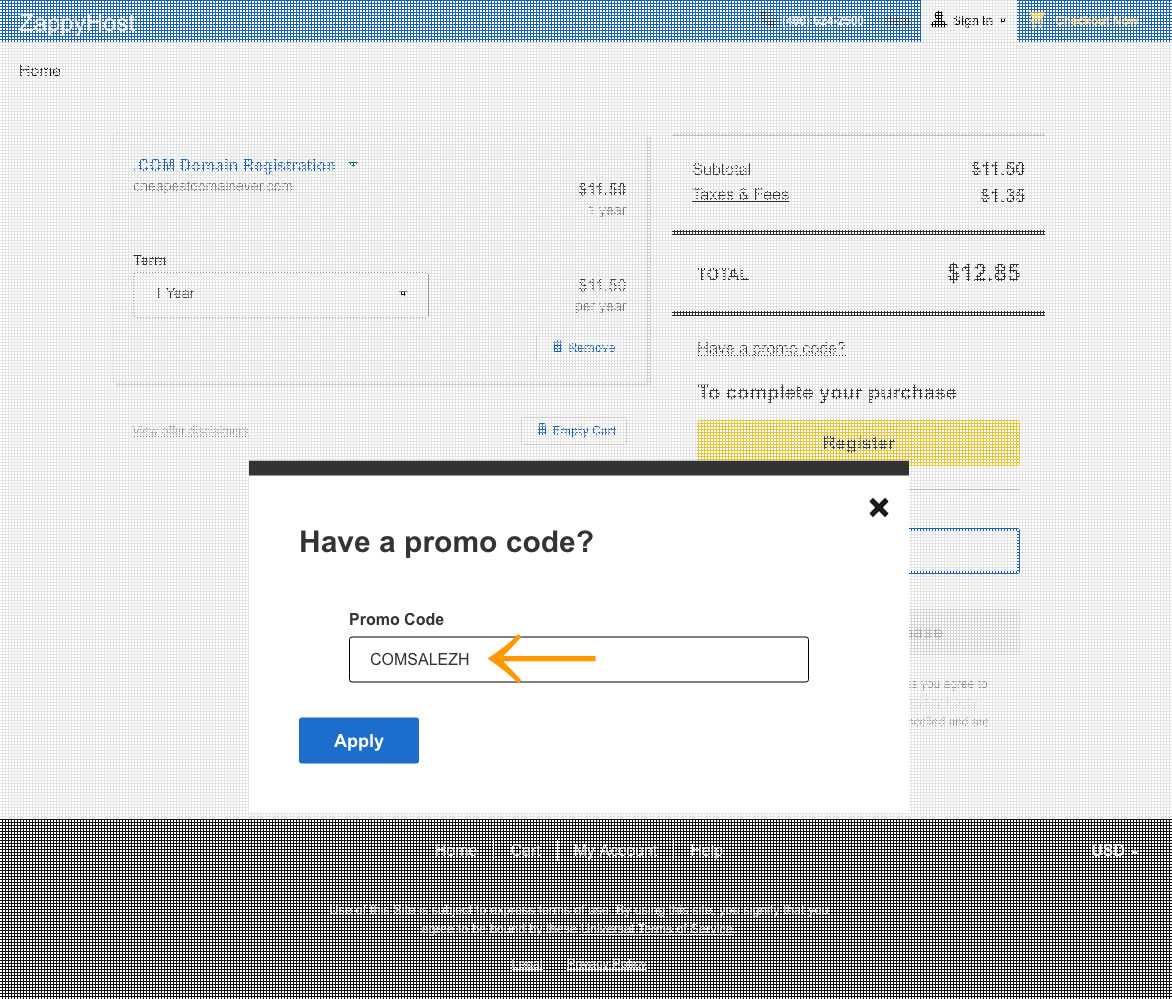The image depicts a domain registration website named "Zappy Host." The background is slightly blurred to focus on a prominent pop-up window in the foreground. The pop-up window has a clean white background with a black rectangular strip at the top, featuring a close button indicated by a black arrow in the top right corner.

The window prominently asks, "Have a promo code?" in bold black text. Just below this question, there is a text box labeled "Promo Code," within which a promotional code, "COMSALEZH," is entered. A dark yellow arrow inside the text box points towards the promo code, indicating its correct placement. Below the text box, a blue tab with the word "Apply" in white is available for users to apply the promo code.

In the blurry background, the website's name, "Zappy Host," is visible in white text on a blue header. Adjacent to it are a sign-in option and a cart icon. Further down, the page details domain registration information. The cost is listed as $11.58 per year with a selected term of one year. The subtotal is displayed as $11.50, with additional taxes and fees amounting to $1.35, making the total $12.85. The phrase "Have a promo code?" appears again, justifying why the promo code window is open.